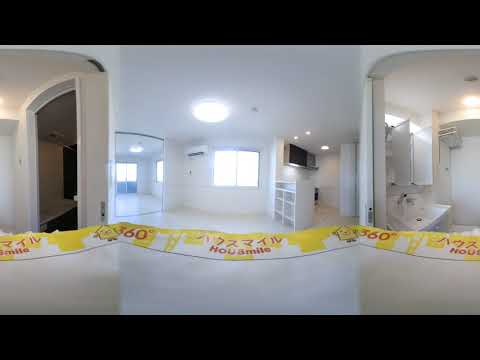The image depicts an indoor scene seemingly stitched together from three fisheye-lens photos. Central to the image is a well-lit white room featuring a large window and a mirror on the left wall. Just right of the window, a small cubby area with a white shelf is visible. Below the window is a yellow and white banner displaying non-English text: "360722TIVNOU8MITE." This banner repeats the number "360" multiple times. On the far left, an arched doorway leads to what might be another interior room, dimly lit and predominantly white. To the right, the image transitions into a pristine, bright white bathroom with a sink, floor, shower stall, and ceiling all uniformly white. Polished floors stretch throughout the scene, enhancing the bright, clean aesthetic. The black border around the top and bottom edges of the image frames the various elements, lending a polished, almost surreal quality to this composite indoor space.